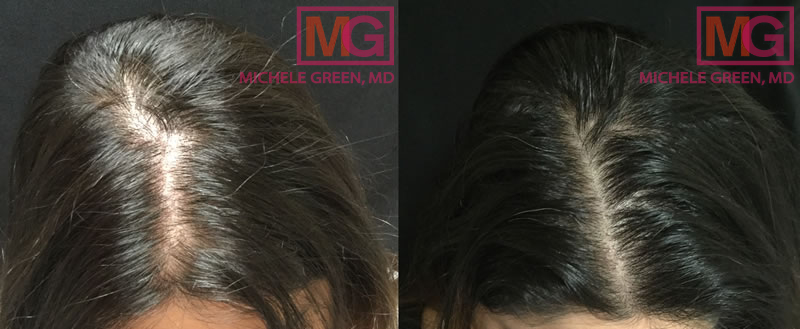This image captures a detailed comparison of hair restoration in a before-and-after format, showcasing the progress of treatment on a woman's scalp identified as Michelle Green, MD. The photograph is horizontally rectangular, comprising two side-by-side square images. Both images focus on the middle part of her head with her dark hair. In the left image, the scalp's part extends from the forehead and curves mid-way, noticeably sparse and revealing a white scalp. Slight graying hairs are faintly visible. The right image depicts the same area post-treatment, where the hair appears fuller, darker, and the part runs straight back, significantly reducing the scalp's visibility. Both images feature a gray background adorned with a logo in the top-left corner; an overlapped capital "MG" in a pink rectangular box, with "Michelle Green, MD" written beneath it in pink letters. Only a small portion of the forehead is visible in both images, emphasizing the focal point on hair density and part characteristics.